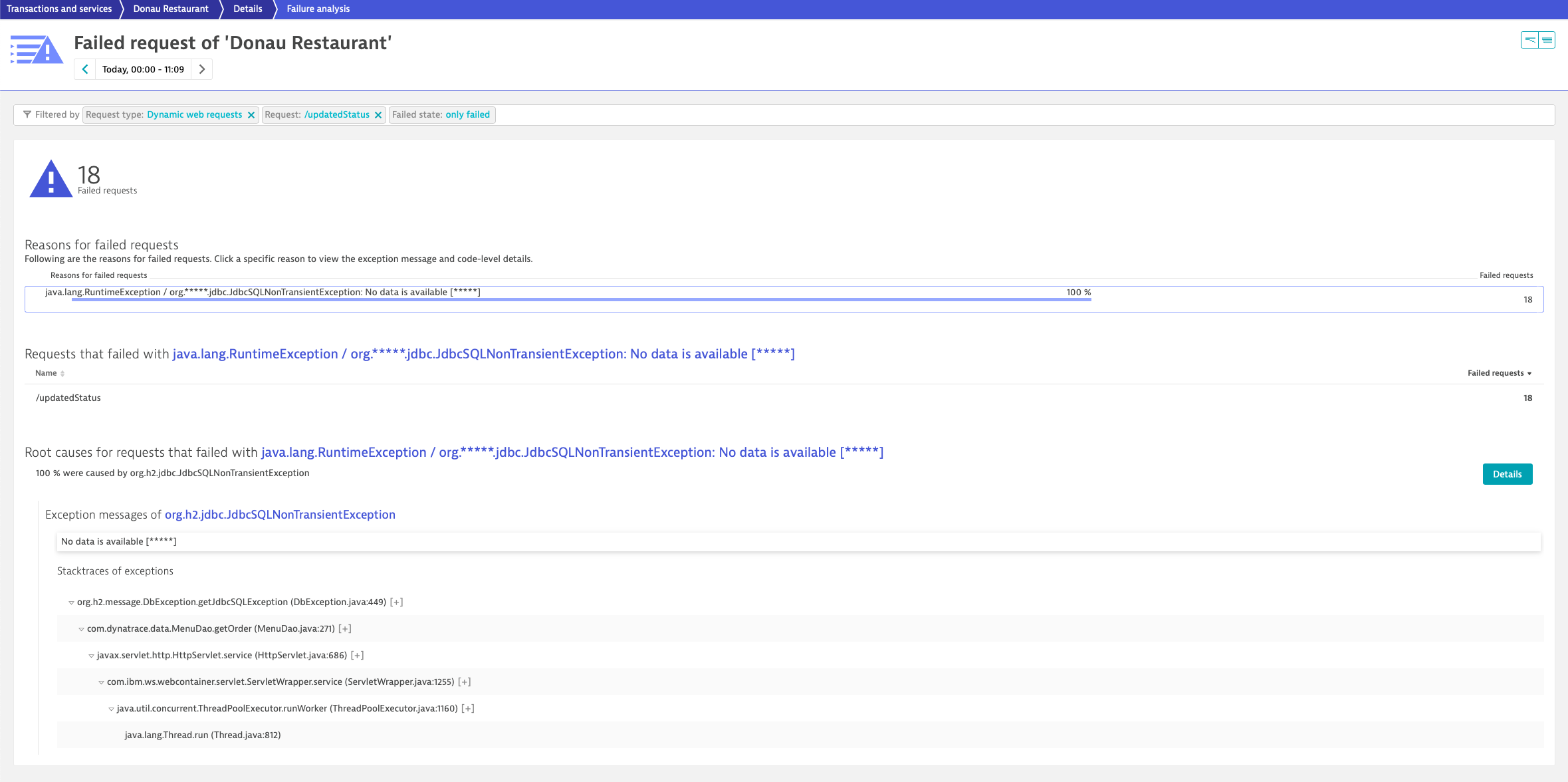This image is a screenshot of a webpage with a white background where much of the text is illegible due to its small font size. At the top, there's a blue border with a left-side menu comprising four items, all written in small white font. In the upper left corner of the page, there is a light blue triangle featuring a white exclamation mark, indicating a warning. Adjacent to this triangle, four horizontal blue lines form a partial square.

Prominently displayed in black font is the message "failed request of a Donau restaurant," with "Donau" spelled D-O-N-A-U. Below this, possibly the word "today" appears, but it is too small to confirm. A thin gray menu strip follows, with sky blue font that's also too small to read.

The main content area beneath the menu continues the white background. Here, a darker royal blue triangle with a white exclamation mark is situated next to a large number "18." Underneath the number 18, the phrase "a failed request" is faintly visible. A headline to the left reads "reasons for failed requests," but the subsequent text is too small to decipher.

Further down, there is a section headed by "request that failed with," followed by a lengthy filename in blue. Below this, another headline states "root causes for requests that failed with," also followed by a long filename. The subsequent lines of text are again too small to be legible.